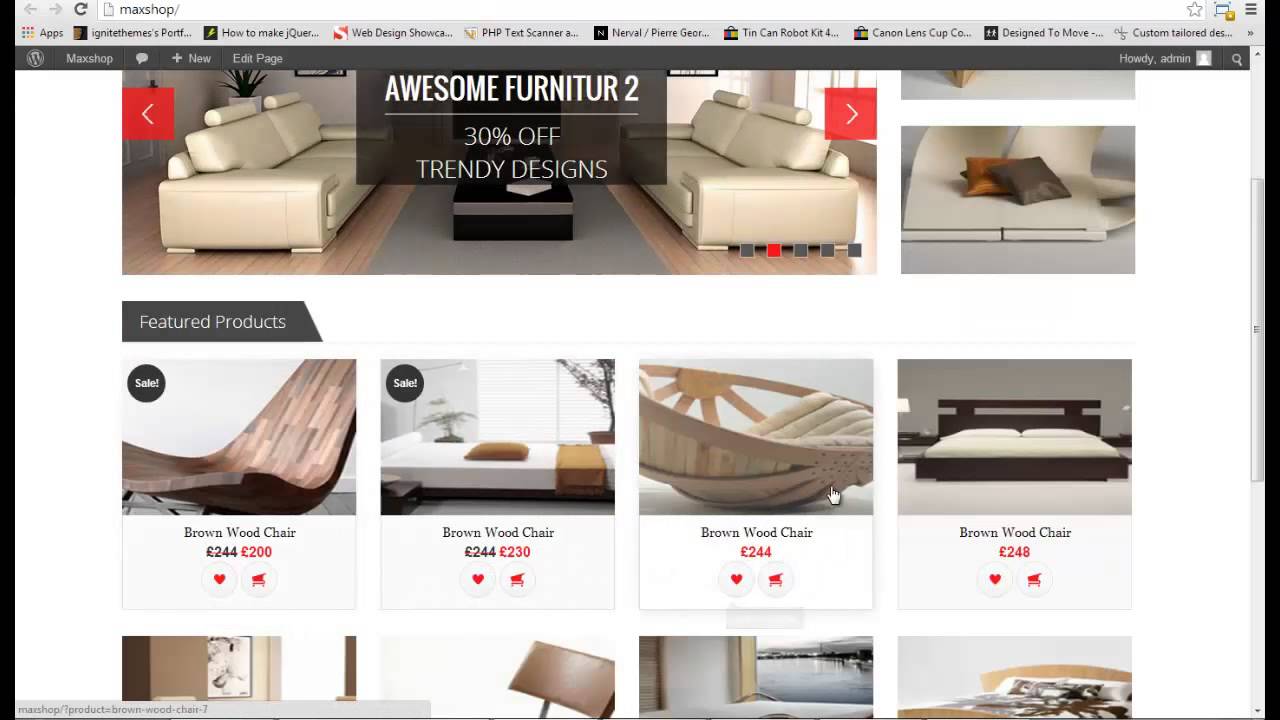The image is a rectangular screenshot of a webpage dedicated to furniture shopping, with the long side oriented horizontally. The webpage is meticulously bordered in black and gray, giving it a clean and structured appearance. At the top, a banner stretches from edge to edge, prominently displaying the text: "Man Shop New Edit Page." Positioned below this banner is a bold promotion, stating "Awesome Furniture - up to 30% off trendy designs."

The background of the page is adorned with various images of stylish furniture pieces. Central to the scene are two couches, artfully arranged to face each other with a chic coffee table sandwiched between them, suggesting a cozy and inviting living area setup. Additionally, there are three distinct brown wood chairs, each featuring unique design elements and individual price tags beneath them.

Along the bottom edge of the webpage, partially visible images hint at a broader range of products such as beds and additional chairs. Enhanced navigation is facilitated by red boxes with white arrows positioned near the couches, allowing users to cycle through the showcased images. On the far right side of the webpage, a scroll bar is available to users, enabling them to explore further furniture options with ease and efficiency.